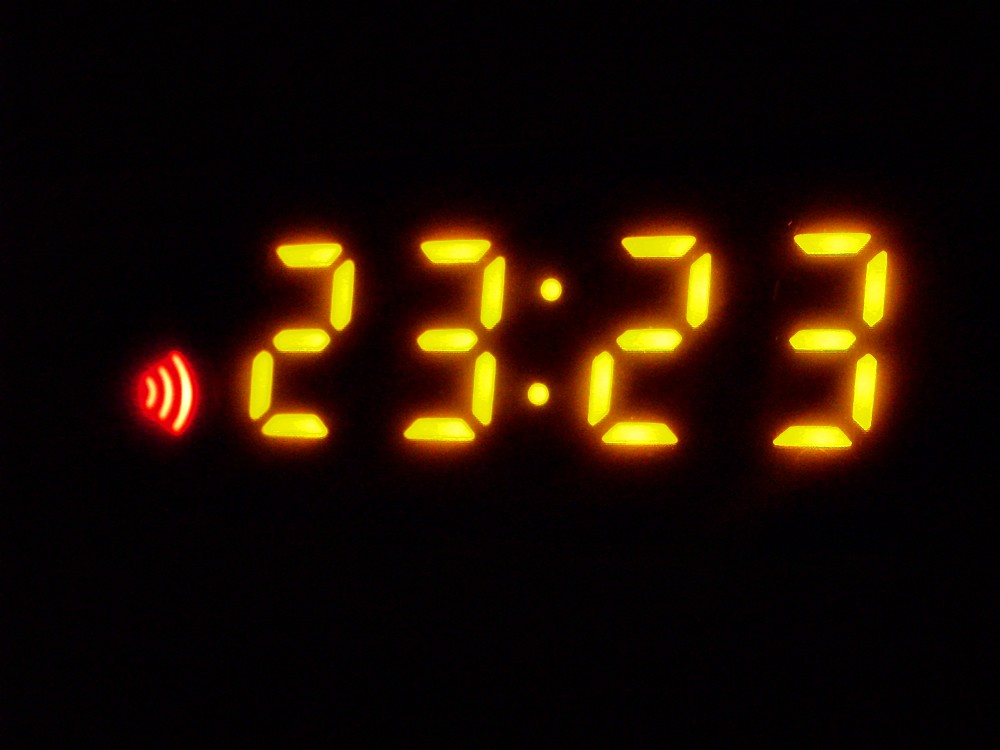This extremely close-up image captures the digital display of an alarm clock. The entire background is pitch black, which contrasts sharply with the bright yellow digital readout. The time displayed is "23:23," formed by bars that constitute each number. To the left of the time, there is a small alarm bell symbol, approximately half the size of the numerals. This symbol has three curved, white bars emanating from it, increasing in size outward, all set against a red background. The yellow numbers have a subtle, brownish-yellow glow or haze surrounding them, enhancing their visibility. Each numeral is constructed of individual bars, such as the number "2" featuring a bar at the top, one on the upper right, one beneath it, another descending on the lower left, and a final bar at the bottom.